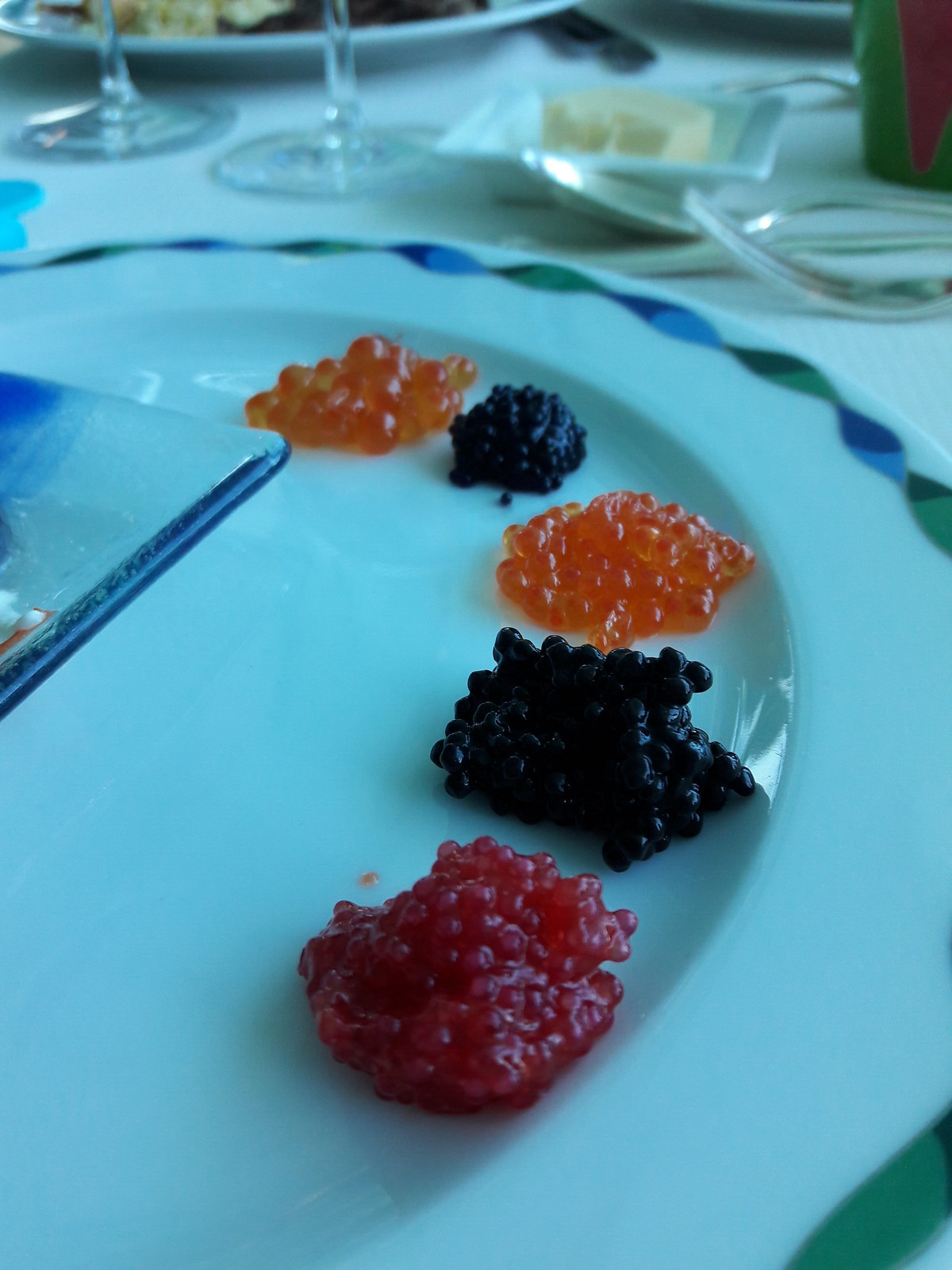This is a close-up color photograph of a white ceramic plate adorned with a decorative trim that includes shades of green, dark blue, and light blue. The plate features five piles of caviar arranged in a slightly curving pattern along its inner edge. The caviar piles are distinctly colored: one red, two black, and two orange. The red and black piles at the front appear larger, each containing at least 75 tiny eggs. In the background, the stems of two wine glasses are visible, along with a small square dish of butter, a plate with some indistinct food on it, and assorted utensils, suggesting a formal table setting. The plate is more vertically oriented, and no text or people are present in the image.